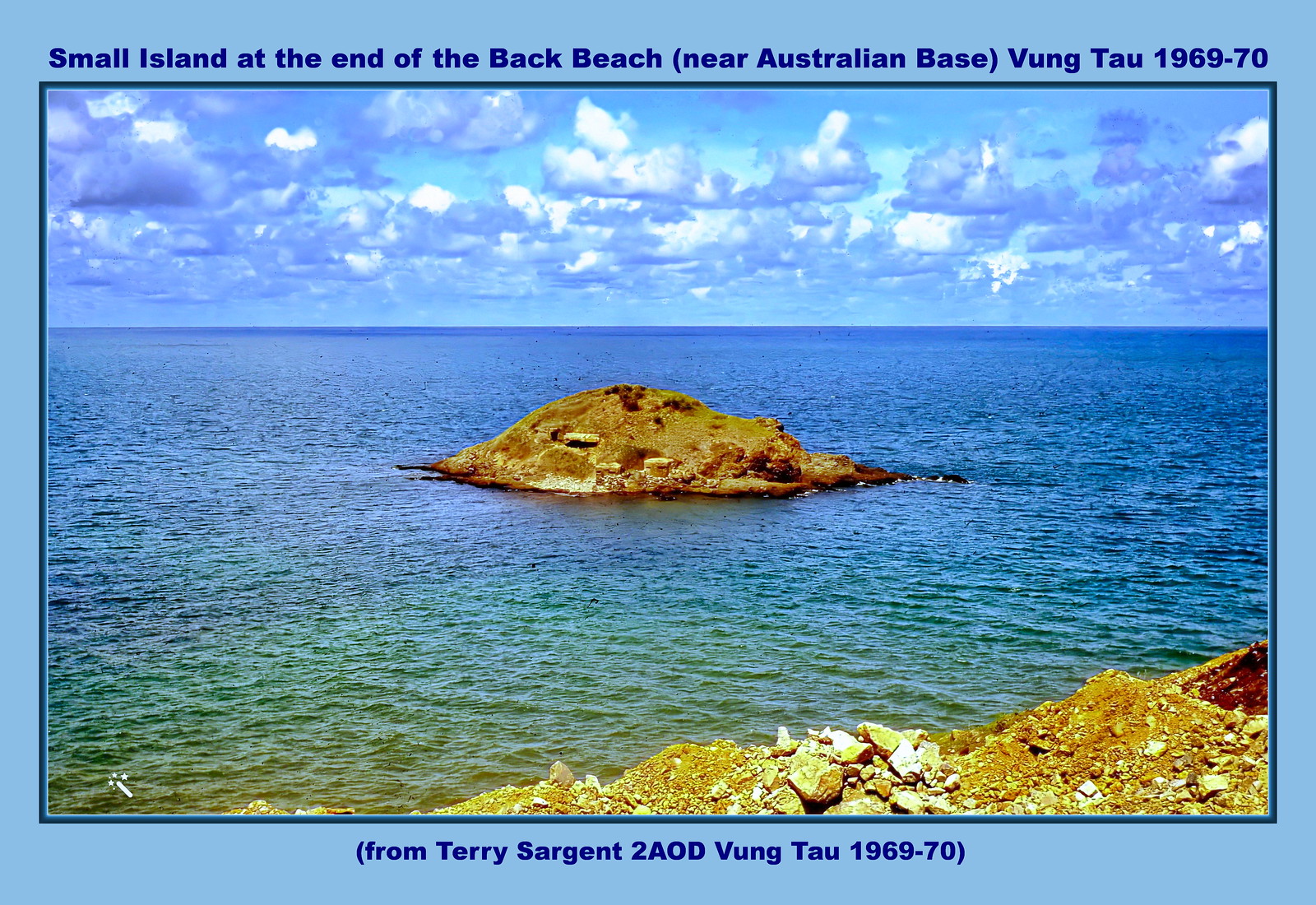This rectangular, postcard-sized photograph, framed in a light blue digital border that is thicker at the top and bottom, captures a serene landscape near the Australian base in Vung Tau, dated 1969 to 1970. The top of the frame reads "Small island at the end of Back Beach (near Australian base), Vung Tau, 1969 to 70" in dark blue font. The bottom of the frame contains the text "(From Terry Sargent to AOD, Vung Tau, 1969 to 70)" in the same color font.

The image predominantly features a body of water transitioning from a blue-green in the foreground to a deeper blue near the horizon. The horizon line is positioned slightly above the center of the photograph. The sky above is populated with cumulus clouds, their lighting exaggerated such that the whites appear blown out and shadows assume an unnatural purple hue. At the center of the water sits a small, uninhabited island, characterized by hues of brownish-green. In the lower right foreground, rocky land with similar brown and green tones is visible. The overall scene portrays a tranquil seascape with slightly rippling waters and a picturesque, cloudy sky.